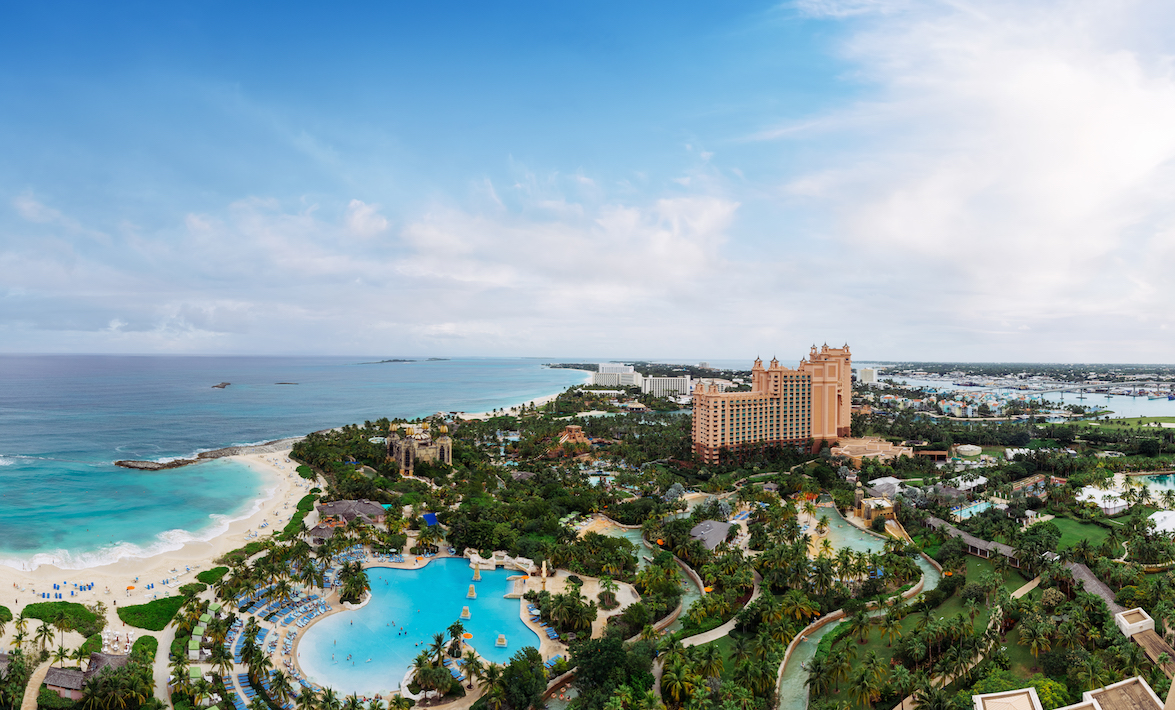The image captures a vivid aerial view of a breathtaking coastal resort. Dominating the center is a tall, multi-story hotel painted in a pinkish beige hue, surrounded by an array of lush greenery and meticulously designed manmade rivers. Directly in front of the hotel, a beautifully inviting pool with light blue water gleams under the sun, accompanied by blue lounge chairs and verdant trees to its left. The scene transitions seamlessly from the manicured green grassy areas and sandy beach to the crystal-clear, bluish-green ocean, which deepens in color as it stretches into the horizon. The sky above is a brilliant blue, adorned with fluffy white clouds, enhancing the serene and paradisiacal ambiance of this waterpark resort nestled near the beach. The entire setting is a picturesque blend of natural beauty and luxurious amenities, making it an ideal seaside escape.